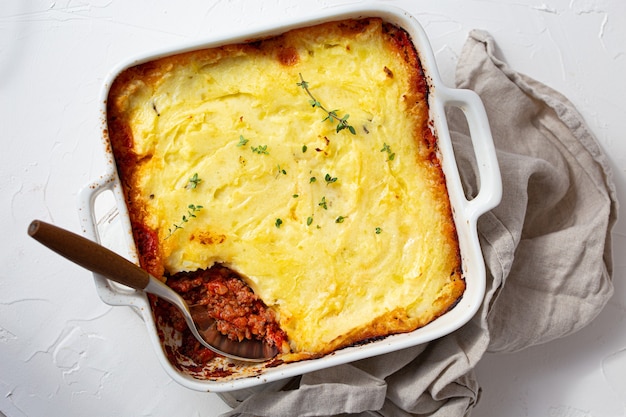The image features a detailed, close-up view from above of a white, square ceramic dish with handles on each side, placed on a grayish napkin resting on a marble surface. Inside the dish is a casserole with slightly charred edges and a gooey, melted cheese topping, sprinkled with green herbs, likely parsley. A silver spoon with a black handle is inserted into the dish in the bottom left-hand corner, revealing a portion of the interior: a mix of ground beef and possibly tomato sauce, showcasing the reddish-brown filling that contrasts with the cheesy top.